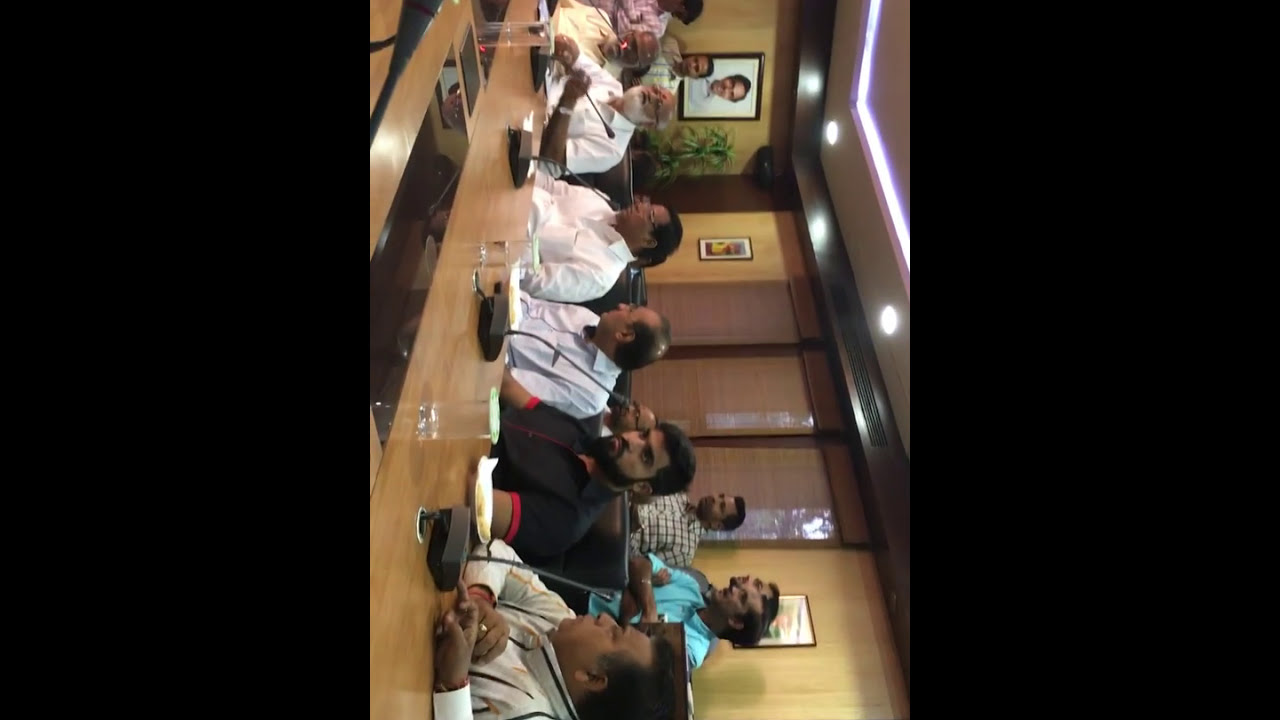This image, oriented incorrectly and requiring a 90-degree tilt to the left for proper viewing, features a rectangular photo inside black borders, capturing a scene indoors with tan walls and wooden doors. At the center of the image, a long rectangular wooden table hosts a panel of six men, all seemingly of Indian or Middle Eastern descent. The men at the table are engaged in an intense discussion, with microphones placed in front of them suggesting a formal meeting, possibly a city council or conference panel.

Prominently, an older gentleman with a bald head and white beard, located near the top of the table, appears to be speaking into a microphone. To his right, a younger man in his 50s with black hair wearing a white long-sleeve business shirt looks on attentively. Another man, also in his 50s with a balding spot, sits next to him, followed by a younger gentleman in his late 30s with black hair and a full beard. The background reveals a few more men standing by the wooden doors, adding to the sense of a crowded and formal setting. The upside-down orientation of the image adds a disorienting effect, making the detailed observation necessary to fully understand the scene depicted.